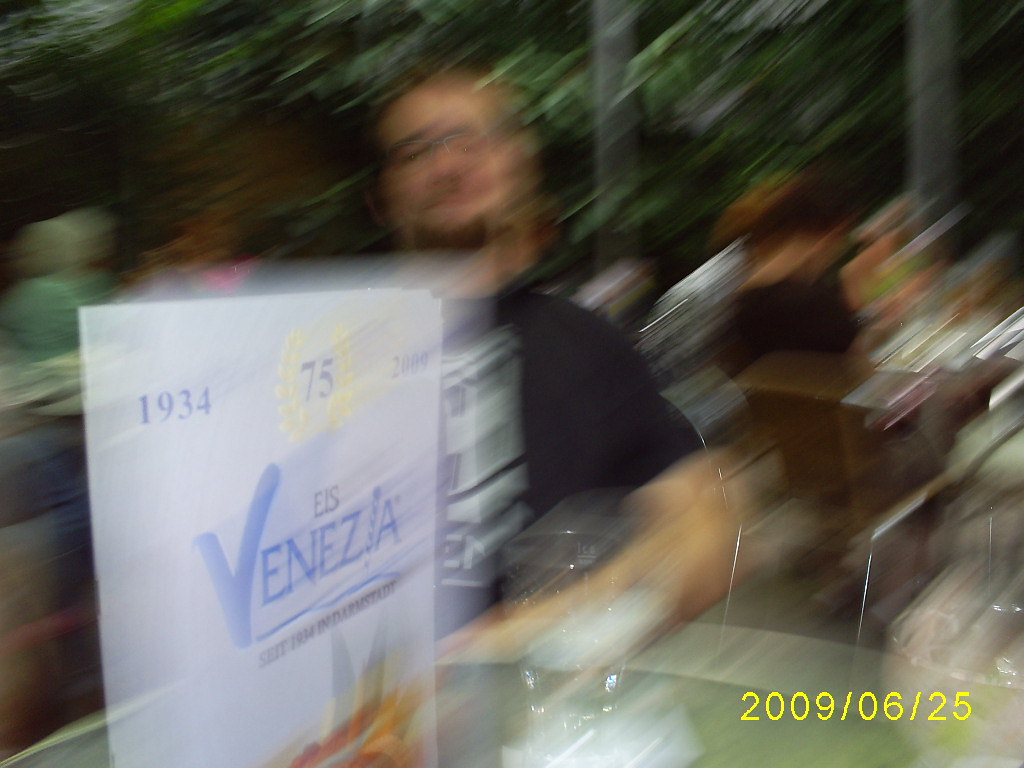The image captures a blurred snapshot of a man sitting at an outdoor restaurant patio. In the background, trees and several tables with other patrons are visible, some of whom are seated wearing various colored shirts. The man in focus, albeit blurred, has brown hair with a balding front, a beard, glasses, and is dressed in a short-sleeved black t-shirt that features a prominent white image on its front. He appears to be smiling while facing the camera. On the table in front of him, a shiny chrome object, potentially the handles of a luggage or chair arms, and a large, upright book or folder can be seen. The book or folder displays a design featuring the text "Venice" or "Ace Venezia," adorned with yellow laurel leaves and marked with the numbers "1934" on the left and "2009" on the right, celebrating its 75th anniversary. A yellow date stamp in the bottom right corner of the photograph reads "2009-06-25."